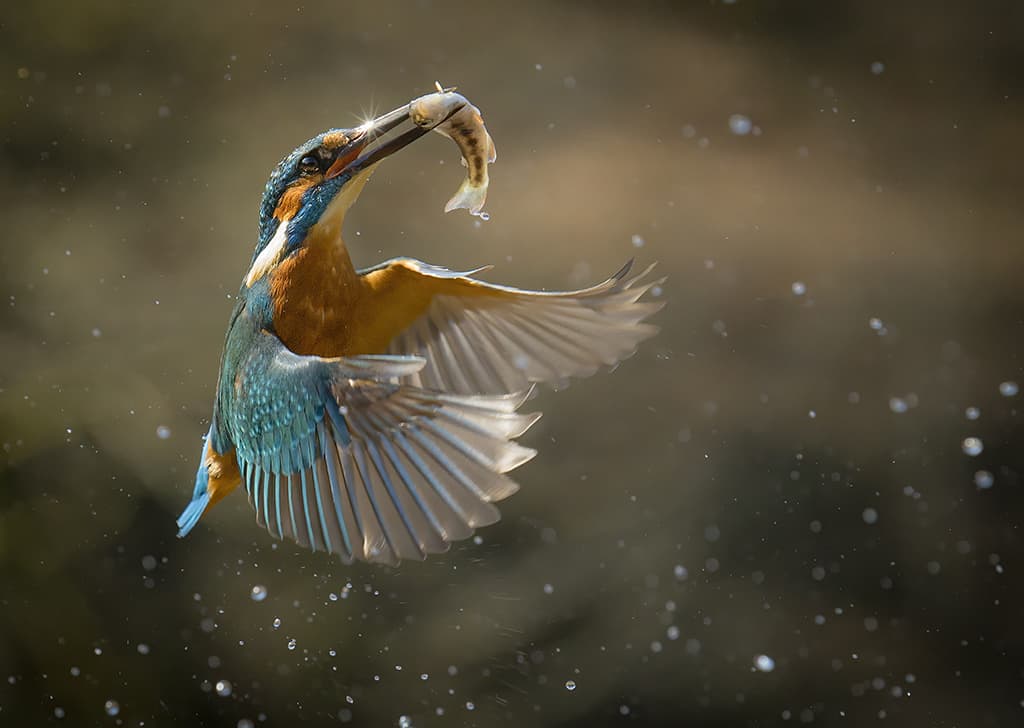In this strikingly detailed AI-generated photograph, a small hummingbird, captured mid-flight, takes center stage. The hummingbird, cloaked in vibrant blue and gold feathers, exhibits an exquisite wingspan with feathers fanned out as it grasps a small, pale orange fish in its long beak. The fish, translucent with a distinct black dotted line through its middle, dangles against the crisp foreground. Watery droplets, suspended in mid-air, suggest the bird has just plucked its prey from a water source below. The bird's chest reveals a blend of yellow and orange hues, with a vivid blue head and orange markings on its cheek. Its gaze, reflecting light, meets the camera directly. The background, beautifully blurred, emphasizes the hummingbird's vivid presence, with the focus slightly off-center to the left. The overall sharpness of the image highlights the intricate details of the scene, from the shimmering water beads to the delicate feathers.